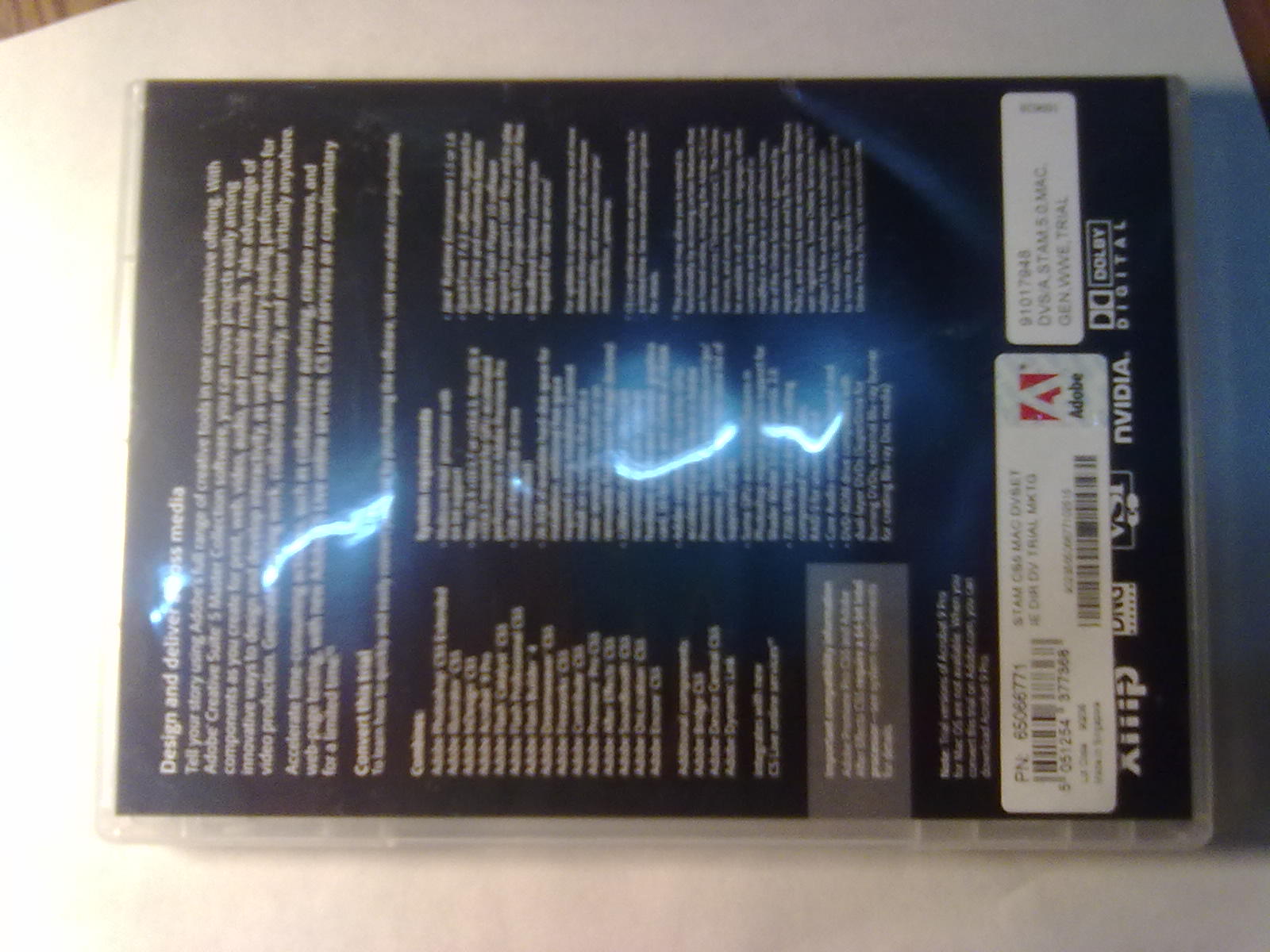The image features a black plastic container, resembling the size of a DVD or games case, placed on a sheet of white printer paper on a wooden table. The container’s back cover is visible and turned 90 degrees to the left, making the white text on it read sideways. The top section of the cover contains a phrase in white text starting with "design and deliver something media" followed by a brief description. Below this, there are three main columns, one of which starts with "contains" and another with "system requirements." The text in these sections is small and difficult to read. At the bottom of the cover, there are two white stickers; one features the Adobe logo— a white 'A' on a red background, accompanied by the text "Adobe" in black, and includes a barcode. The other sticker displays additional numeric information. Additional logos, including NVIDIA and Dolby Digital, are also present. A glare from bright blue lights is visible against the white background surrounding the box, adding an illuminated effect to the image.